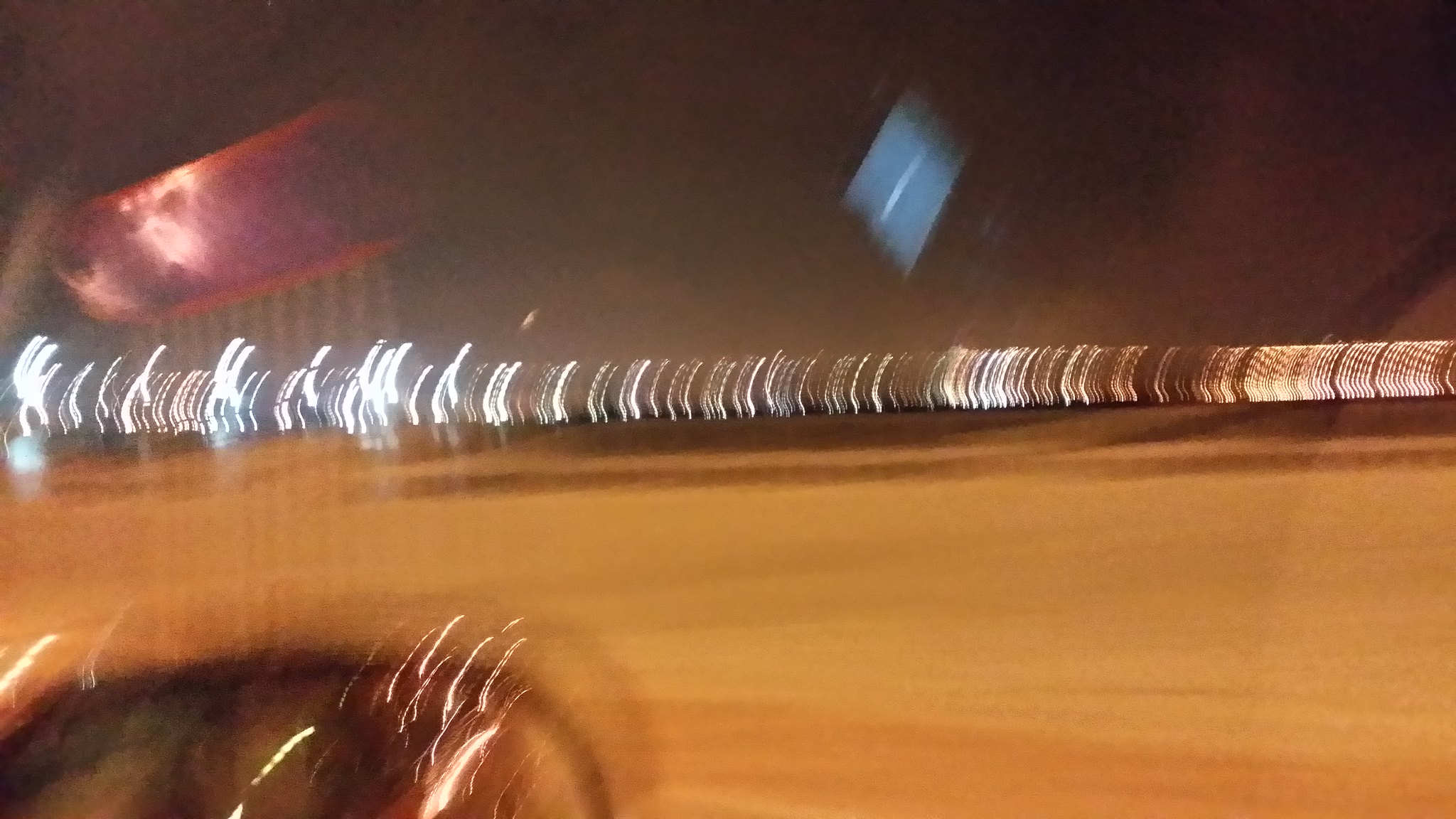An outdoor color photograph taken at nighttime from the right side of a moving vehicle. The image is heavily blurred, capturing a horizontal string of lights running from the center left to the center right of the frame. These lights appear as vertical streaks that are slightly convex to the right. In the lower left corner, the right rearview mirror of the car is visible, reflecting some light. The background below the lights is a tan-hued area, possibly a roadway or sidewalk, with light pollution haze adding a glow above the lights. Upper portions of the image are dark, but feature a red, almost pink, oval light to the left and a blue diamond-shaped light on the right, both blurred reflections possibly from inside the vehicle or signs in the distance.